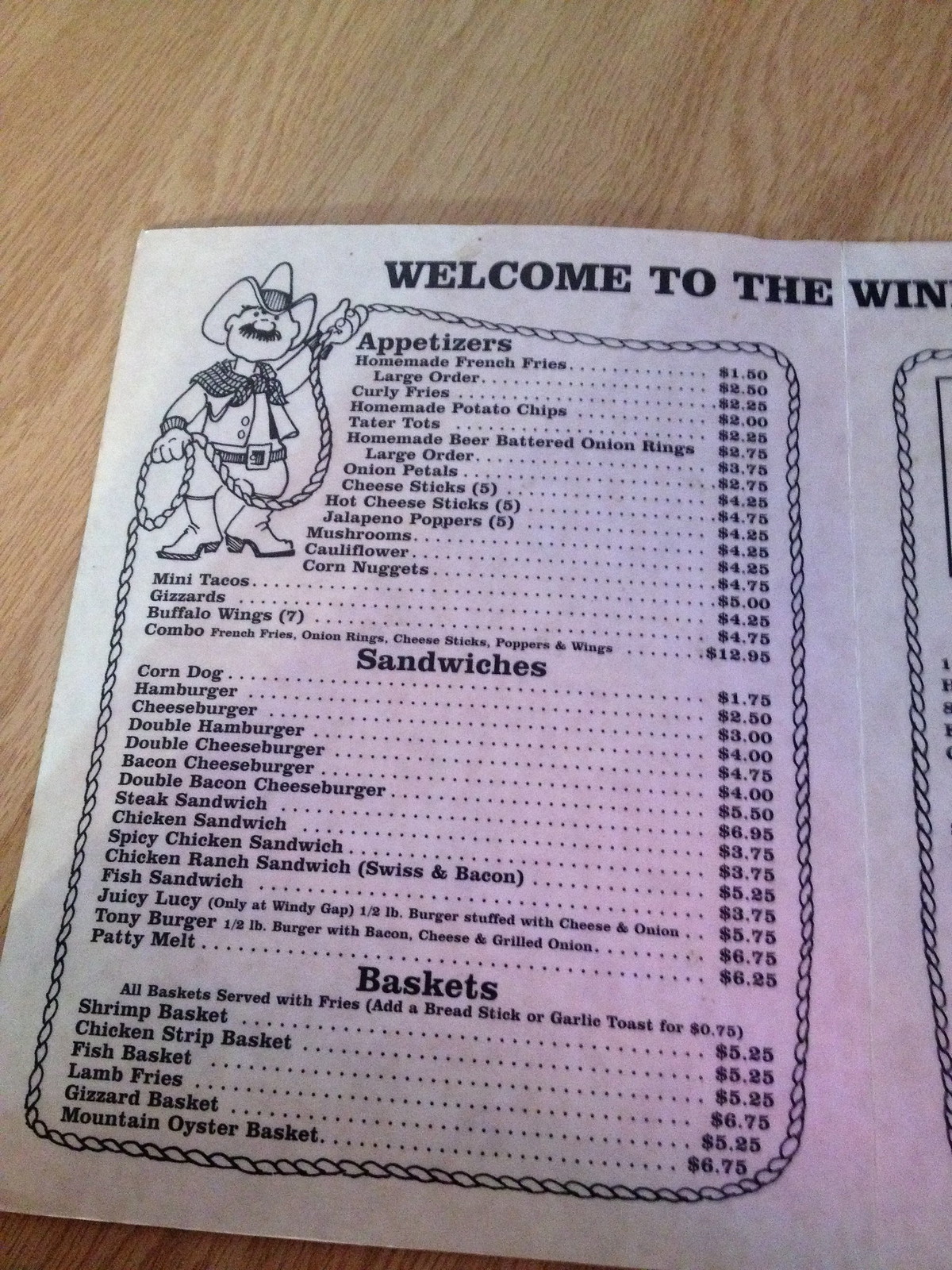A white menu sits on a rustic wooden table, displaying the upper left half titled "Welcome to the WIN." The focal point is a whimsical drawing of a cowboy in the upper left-hand corner. He's adorned with a 10-gallon hat, prominent mustache, vest, scarf, black belt, and cowboy boots. The cowboy grips a coiled rope in his right hand, while his left hand is raised as the rope weaves around the menu, artistically framing the offerings. The menu features sections for appetizers, sandwiches, and baskets, listing items priced from $1.50 up to $6.75. The cowboy's rope envelops these sections, providing a unique presentation that captures the rustic western theme of the restaurant.